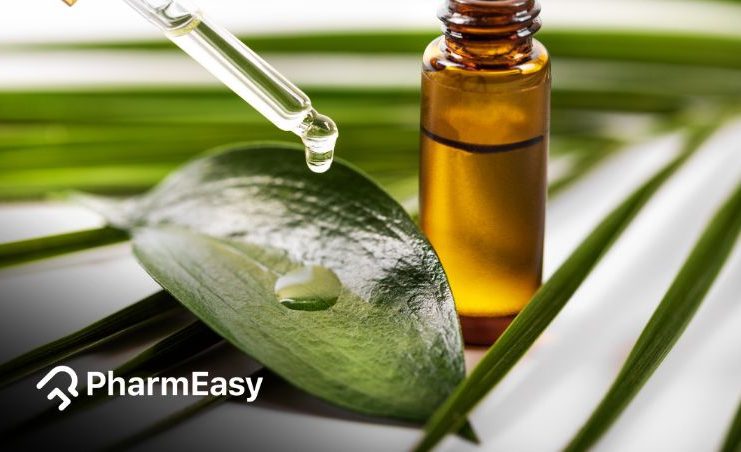This detailed color photograph, in landscape orientation, captures a close-up scene of a tea tree oil dropper and an amber-colored vial against a white surface. At the center, a shiny, green leaf with a glassy texture is angled from the top left to the bottom right, featuring a small hole. A dropper, entering the image from the top left, releases a clear droplet of tea tree oil onto the leaf, while another droplet hangs poised to fall. To the right of the leaf stands a small, vertical amber vial filled three-quarters with a clear liquid, cropped at the screw-top opening. The background, slightly out of focus, features thin bands of leaves, notably a palm frond. In the bottom left corner is the bold white text "PHARM Easy" alongside the P-E logo, linking the image to the Farm Easy brand. The photograph, styled in representational realism, emphasizes the leaf's reflective surface and intricate details, framed by the surrounding greenery.